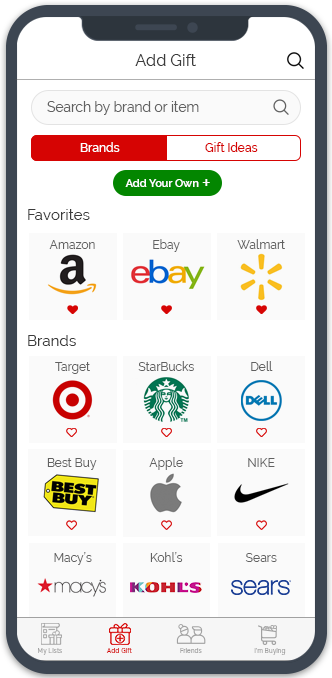The image depicts a cell phone screen showing a gift-giving app interface. At the top, there is an "Add Gift" option accompanied by a magnifying glass icon for search functionality. The search bar below reads "Search by brand or item" with an additional search icon, offering selections for "Brands" or "Gift Ideas." Centrally positioned beneath the search bar lies a prominent green button labeled "Add Your Own" with a white plus sign.

The screen's lower section is organized into various categories. Under "Favorites," the app displays icons for Amazon, eBay, and Walmart, each accompanied by their respective logos (Amazon's signature smile, eBay's multicolored lettering with 'E' in red, 'B' in blue, 'A' in yellow, and 'Y' in green, and Walmart's yellow spark). These icons are marked with solid heart icons, indicating they have been selected as favorites.

Below the "Favorites" section, the "Brands" category lists several brands with their logos: Target (red and white target symbol), Starbucks (green siren logo), Dell (Dell's distinctive font), Best Buy (yellow price tag logo), Apple (silver apple), Nike (black swoosh), Macy's (red star), Kohl's (stylized text), and Sears (classic Sears logo). In this section, the Target icon has a heart that is not solid, indicating it is not yet marked as a favorite. At the screen's bottom, navigation icons read "My Lists," "Add Gifts," "Friends," and "I'm Buying," helping users to easily navigate through the app's features.